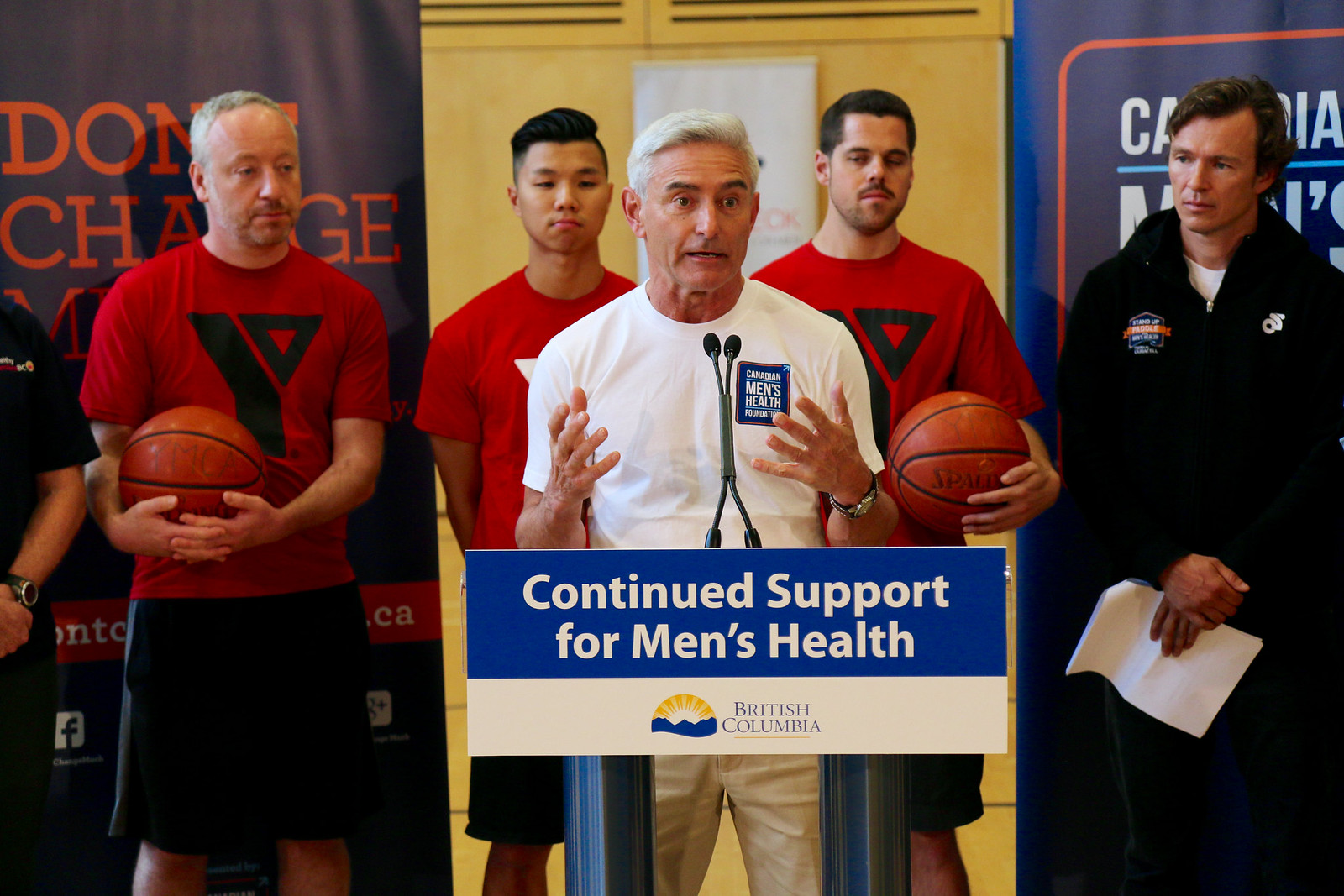In the image, an older, fit man, likely in his 50s or 60s with gray hair, stands at a podium giving a speech. He is dressed in a white t-shirt emblazoned with "Men's Health" on the chest and paired with off-white or khaki trousers. The podium has a blue and white sign that reads "Continue Support for Men's Health" with a subtext in grey saying "British Columbia," accompanied by a rising sun behind a mountain logo.

Flanking the speaker are several men. Two men are wearing red t-shirts with YMCA logos, each holding an orange basketball with black stripes, and dressed in black shorts. One of them is bearded, and another has short white hair and a French beard. To the right, a person dressed in a black half-zip jacket over a white t-shirt and dark blue pants stands with some emblems on their jacket. Another individual, partly visible, is in a black hoodie with the "Stand Up With Miracle" logo and ribbon, and is holding a piece of paper.

Behind the group, a yellow wall serves as a backdrop adorned with various banners. One banner has bold orange letters stating "Don't Change M," along with partially visible text in a red strip and icons for Facebook and Google+. The scene suggests a community or motivational event focused on men's health, involving representatives from the YMCA and other local organizations.